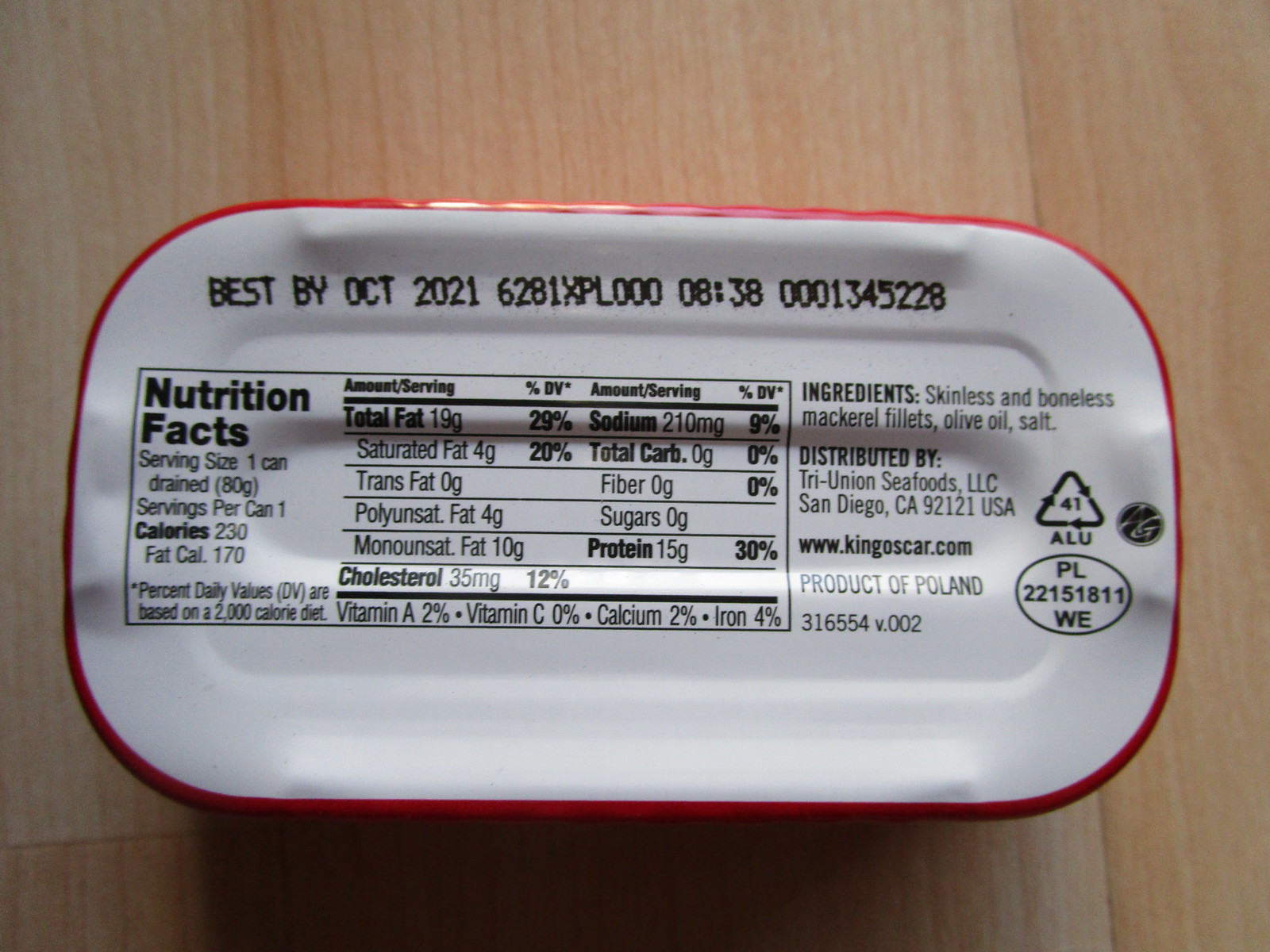The image shows the bottom of a tin of skinless and boneless mackerel fillets. The can features a white background with a red rim around the edge, and it is set on a light brown wooden surface. All text is printed in black. At the top, it reads "Best by Oct 2021 6281XPL000 08:38 0001345228." Below this, there is a standard nutrition facts box detailing the following: serving size 1 can drained 80 grams, servings per can 1, calories 230, fat calories 170, total fat 19 grams, saturated fat 4 grams, trans fat 0 grams, polyunsaturated fat 4 grams, monounsaturated fat 10 grams, cholesterol 35 milligrams, sodium 210 milligrams, total carbs 0 grams, fiber 0 grams, sugar 0 grams, protein 15 grams, vitamin A 2%, vitamin C 0%, calcium 2%, iron 3%. To the right of the nutrition facts box is the ingredients list: skinless and boneless mackerel fillets, olive oil, salt. Further details indicate it is distributed by Tri-Union Seafoods LLC, San Diego, California, 92121 USA, with a website www.kingoscar.com. It is marked as a product of Poland with a code 316554 version .002. There is a recycling symbol with the number 41 in it, labeled "ALU," followed by an oval with "PL22151811" and below that "WE."